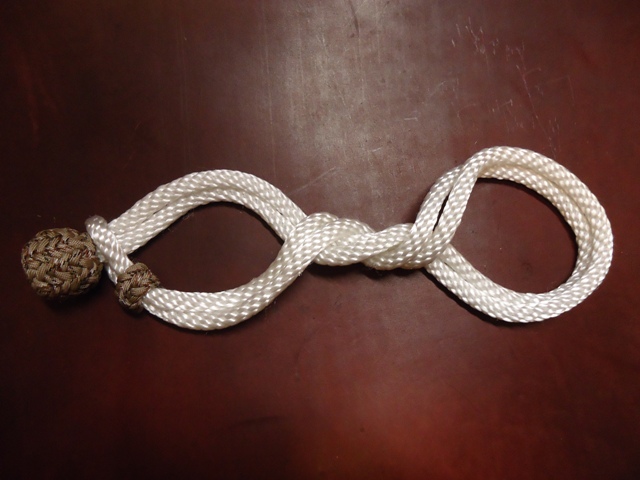The detailed image showcases a bright white rope intricately tied and knotted, resting on a dark reddish-brown wooden surface that appears almost like leather. The rope's central section twists to create a double-loop resembling an infinity symbol or a pair of eyeglasses, with each loop facing opposite directions. Near the left side, a large brown knotted area or knob interlocks with another part of the rope, securing it in place. The rope itself forms one long continuous piece, and the bright knot contrasts sharply with the dark wooden table. The surface features a subtle gradient of color, lighter at the center where light falls, producing a striking visual effect against the darker corners. This convergence of textures and shapes creates a detailed, almost tactile depiction of the rope and its elegant knots.